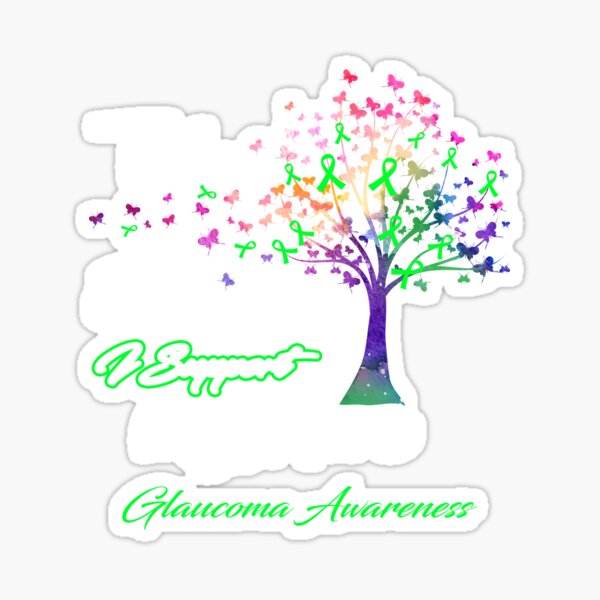The image depicts a stylized, 2D illustration of a tree as the emblem for a glaucoma awareness charity or support group. The tree, set against a pristine white background, combines elements of a rainbow and galactic aesthetic, with a base in green seamlessly blending into a purple trunk, culminating in a burst of vivid, multicolored branches. These branches are adorned with predominant green ribbon bows in various sizes, symbolizing awareness, while an array of pink, red, and orange butterflies, some faintly depicted, flutter around the top and left side of the tree. The image is framed by a simple gray border. Below the tree, in large green lettering with white interiors, the phrase "I support" is prominently featured. Beneath this, in a connected section, also in green, the words "glaucoma awareness" are displayed. The overall design conveys a message of support and awareness for glaucoma.